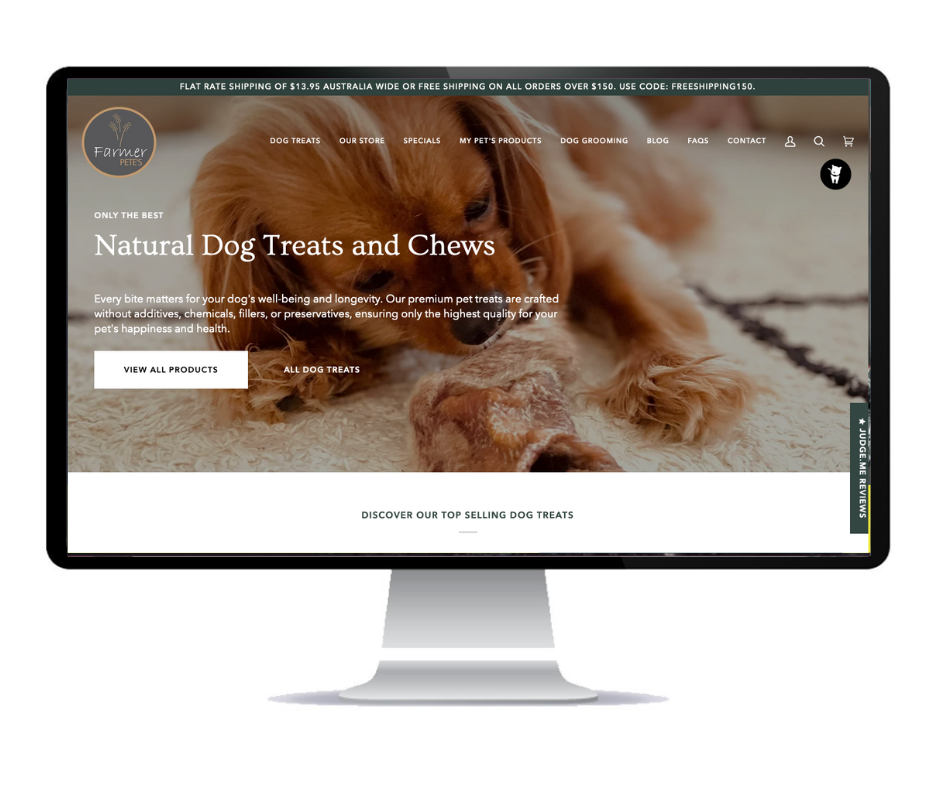The image resembles the shape of a computer monitor, complete with a white stand at the bottom, suggesting it is standing on a surface. The monitor screen itself features a black border, and is displaying a website.

The website appears to be either "Farmer Pets" or "Farmer Pete’s," as deciphered from the slightly unclear text. The logo is positioned in the upper left corner, depicting a circle with yellow dashes, and the words "Farmer" in white and "Pete's" in yellow.

Across the top of the screen, a notice bar reads: "Flat Rate Shipping $13.95 Australia Wide or Free Shipping on All Orders Over $150, Use Code FREESHIPPING150." Below this are menu options, centered and listed in white text, including: Dog Treats, Our Store, Specials, My Pets, Products, Dog Grooming, Blog, FAQs, and Contact. There is a small black circle icon with a white cat within it, perhaps indicating a clickable link or menu option.

Below the menu, text reads: "Only The Best Natural Dog Treats and Chews. Every bite matters for your dog's wellbeing and longevity. Our premium pet treats are crafted without additives, chemicals, fillers, or preservatives, ensuring only the highest quality for your pet's happiness and health."

A white button underneath this text says “View All Products” in black lettering, next to which is additional text in white indicating “All Dog Treats.” At the very bottom, a thick white bar extends across the width of the screen, inviting viewers to "Discover Our Top Selling Dog Treats."

The background image, apart from this white bar, showcases a photograph of an adorable puppy lying on a rug, fixated on a fuzzy toy on the ground. This charming, playful scene enhances the overall appeal of the website.